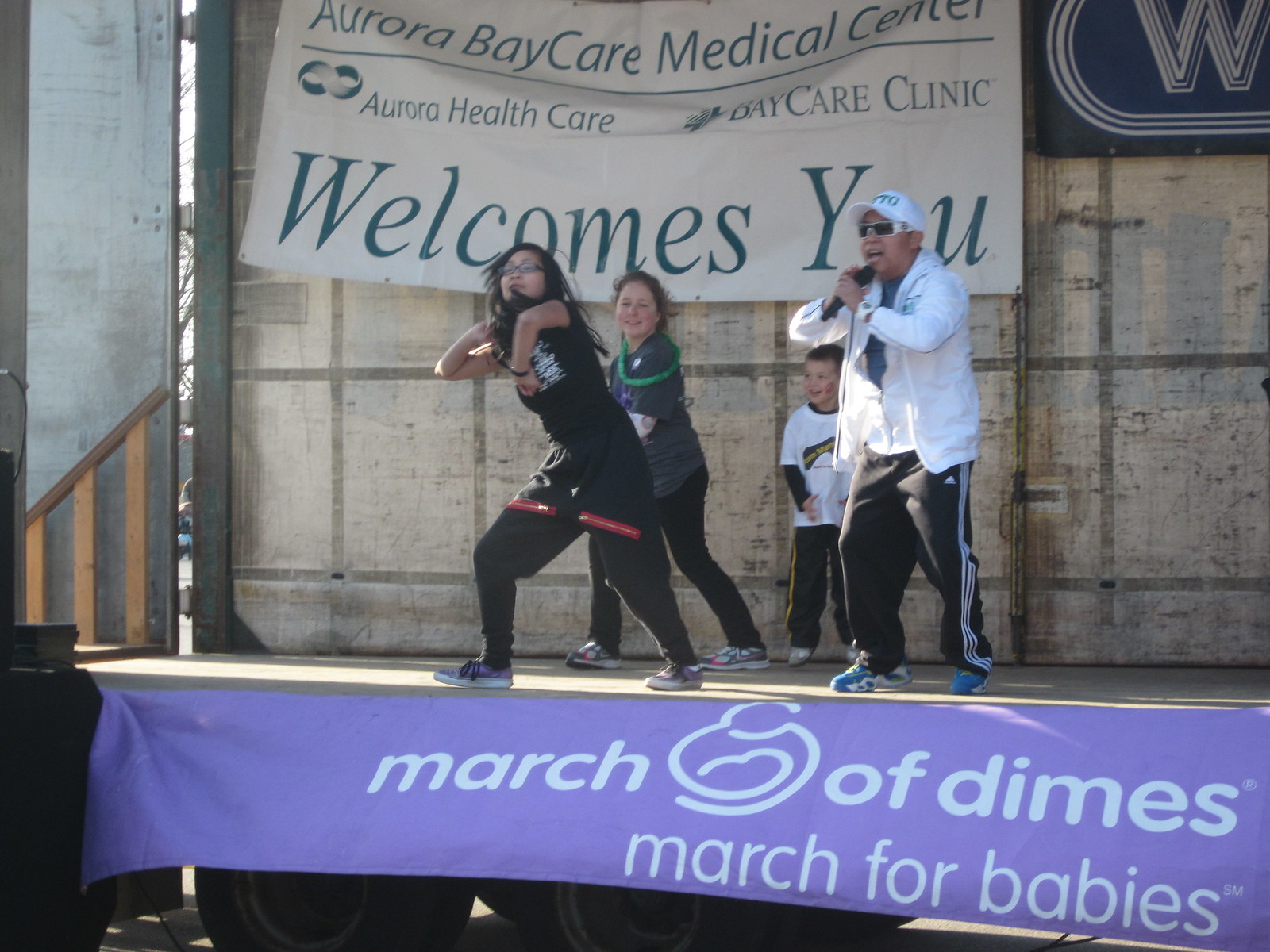A vibrant family performance is unfolding on stage, conveying joy and unity. At the top left corner, a sign reads "Aurora BayCare Medical Center, Aurora Healthcare, Daycare Clinic welcomes you," suggesting the event is hosted by these healthcare organizations. In the top right, a prominent "W" is visible. 

On stage, a man dressed in a white hoodie and black pants passionately sings into a microphone. Behind him, three children are energetically dancing: a little boy wearing a white shirt and black pants, a girl in a bluish shirt and black pants, and another girl in a black shirt and black pants. Below the performers, text reads "March of Dimes, March for Babies" accompanied by a purple banner with white lettering at the bottom of the stage, highlighting the charitable cause of the event.